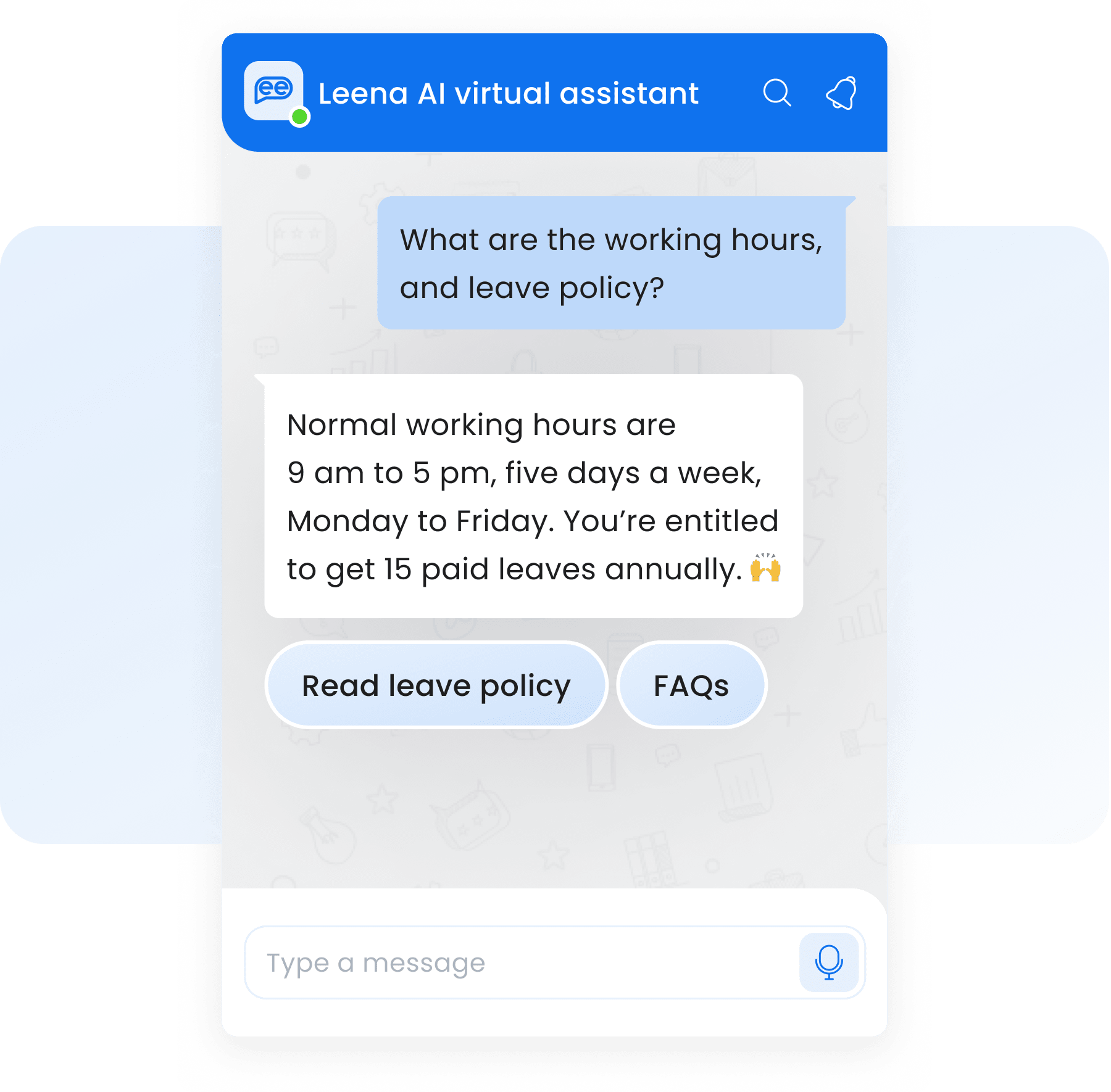The screenshot captures a lively conversation on a computer screen between a user and Lina, an AI-powered virtual assistant. At the top of the chat interface, a small icon labeled "EE" represents Lina, who has just received a query about work-related policies. The search bar and notification bell icon are visibly positioned for easy access.

In the dialogue, Lina responds to a user's question about the working hours and leave policy, which is presented in a light blue chat bubble: "What are the working hours and leave policy?" Lina's reply, displayed in a white bubble, states, "Normal working hours are 9 a.m. to 5 p.m., five days a week, Monday to Friday. You are entitled to 15 paid leaves annually, equivalent to three weeks." The message is punctuated with a clapping hand emoji, adding a friendly touch.

Beneath this, a blue chat bubble provides additional links labeled "Read Leave Policy" and "FAQs," suggesting that these are attachments or further resources the user can click on for more detailed information. The interface also features a text input field at the bottom, along with a button allowing the user to voice their queries. This setup indicates an interactive AI system designed to assist the user with job-related inquiries efficiently.